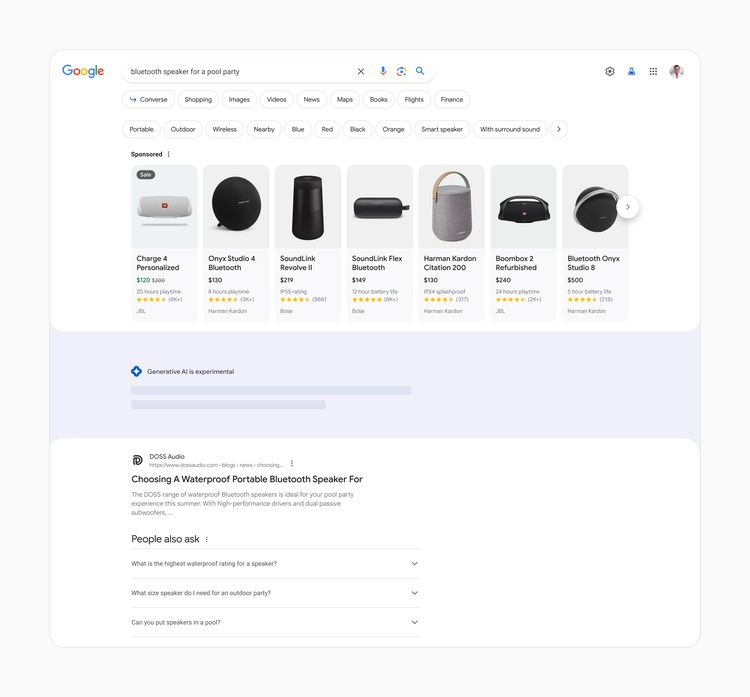A user has searched for "Bluetooth speaker for a pool party" on Google, resulting in a diverse selection of options. The search results display a variety of portable Bluetooth speakers with different features and price ranges. Among the highlighted options are:

- JBL Charge 4, which is noted as personalized.
- Harman Kardon Onyx Studio 4, another Bluetooth speaker option.
- Bose SoundLink Revolve, alongside the Bose SoundLink Flex.
- A more expensive Harman Kardon model, acclaimed for its speaker quality.
- A refurbished JBL Boombox 2.
- Harman Kardon Onyx Studio 8, which appears to be the most expensive among the listed options.

Beneath the search results, there's a disclaimer noting that "Generative AI is experimental," marked with a blue insignia. This section is designed to be helpful in choosing a waterproof portable Bluetooth speaker. Additionally, the "People Also Ask" section offers common queries such as, "What is the highest waterproof rating for a speaker?" This helps users gather more information to make an informed decision.